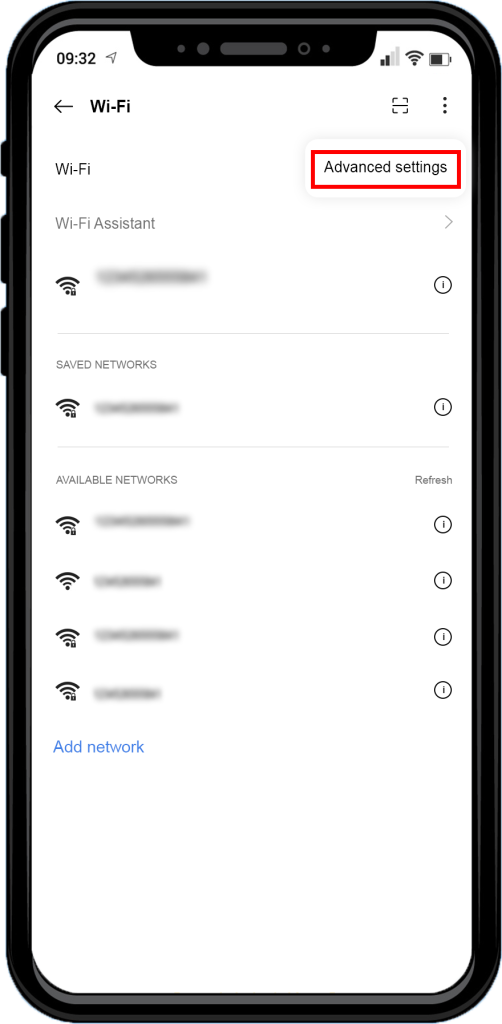The image shows a black-cased cell phone, which stands about two and a half to three times taller than it is wide. On the left side of the phone, there are three buttons: a small one at the top followed by two larger ones. The phone's screen displays detailed information related to Wi-Fi settings.

In the upper left corner of the screen, the time reads 9:32. The upper right corner displays the Wi-Fi signal, cellular signal strength, and battery life indicators. Below this, the screen presents a user interface for Wi-Fi settings.

On the left of this interface, there is a back arrow icon, followed by the title "Wi-Fi." To the right, there are icons for a square and a menu. Directly below the "Wi-Fi" header, a red rectangle highlights the "Advanced settings" button, which sits to the right of the Wi-Fi label.

Further down, the "Wi-Fi assistant" is shown but grayed out, with a grey arrow on the right side. The next section displays the current Wi-Fi connection. Although the name of the network is blurred out, the signal icon appears on the left.

Below the current connection, there is a section for saved networks, followed by a list of available networks at the bottom of the screen. The detailed interface and highlighted settings suggest the image is focused on guiding the user through Wi-Fi configuration options.